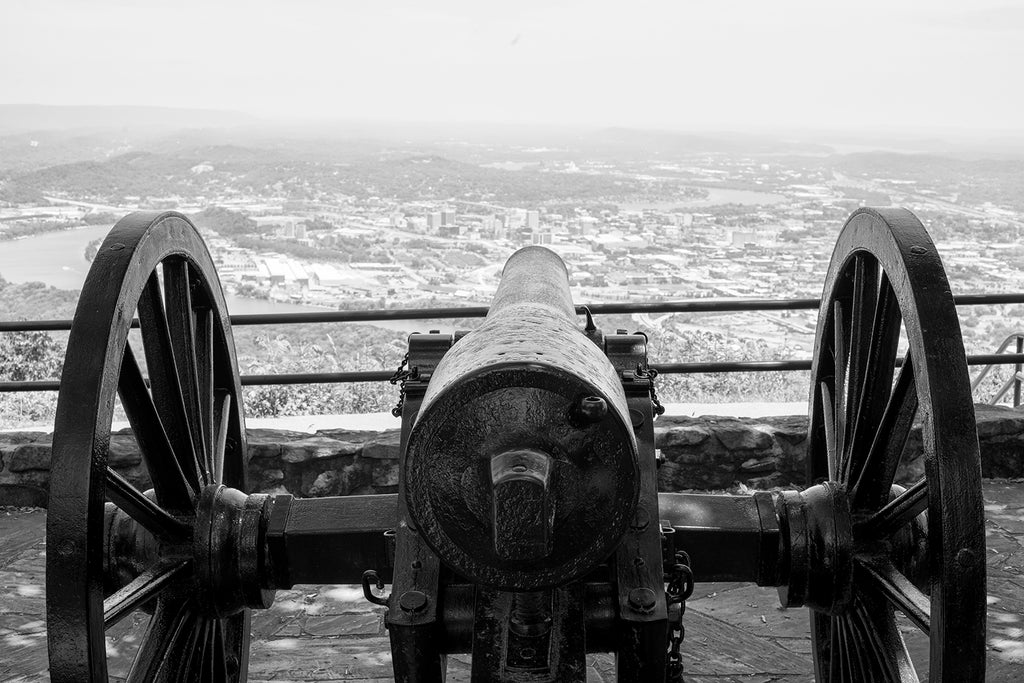This black and white photograph, taken outdoors, captures a serene and historically significant scene. Featuring a Civil War-era cannon from behind, the photo zeroes in on the iron cannon supported by two large wooden spoke wheels on either side. The cannon is set atop a stone surface, overlooking a metal railing with a small stone step. Beyond this railing lies a city sprawling across a basin, with a river cutting through its outskirts on the left and meandering towards the center. The setting appears to be a historical site, possibly a fortification on a hillside, where the cannon once stood guard. The scene is shrouded in a light gray haze, indicative of a foggy or smoggy day, adding a layer of mystique to the morning landscape. The photograph captures an interplay of historical elements and natural beauty, offering a glimpse into a bygone era against the backdrop of a tranquil, foggy cityscape.